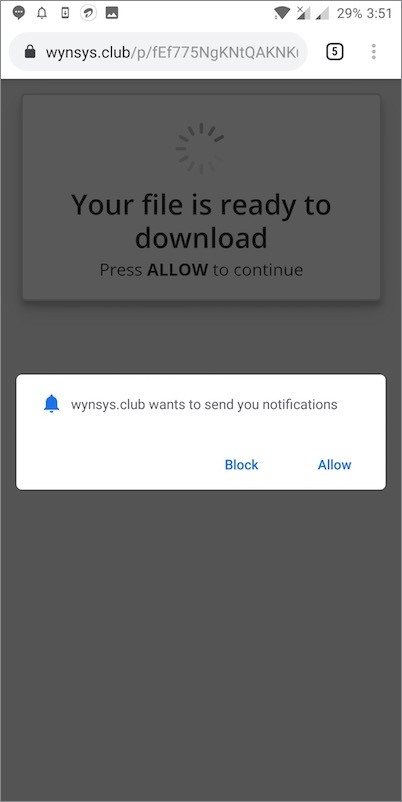Screenshot from a smartphone web browser displaying a notification prompt. The header bar, featuring a white background, contains two rows of icons. The first row includes icons such as a generic messaging symbol, a bell likely representing notifications, a smartphone icon with a down arrow, a stylized letter "D," and a landscape mode image icon. On the right of the first row, there's a Wi-Fi signal indicator, a signal strength indicator halfway filled with an "X," another signal indicator partially filled, a battery indicator showing 29%, and the time noted as 3:51.

The second row shows a truncated web address displayed in black text on a grey box. To the right of this, a number "5" indicates five open tabs, followed by a contextual menu represented by three grey dots. Dominating the screenshot is a central dialog box with a white background and grey overlay on the rest of the screen. The dialog box, from W-I-N-S-Y-S.club, is asking permission to send notifications, indicated by dark grey text and a blue bell icon. Below, there are options to "Block" or "Allow" the request in blue. Additionally, the dialog overlay includes text stating "Your file is ready to download, press allow to continue" and a throbbing progress indicator.